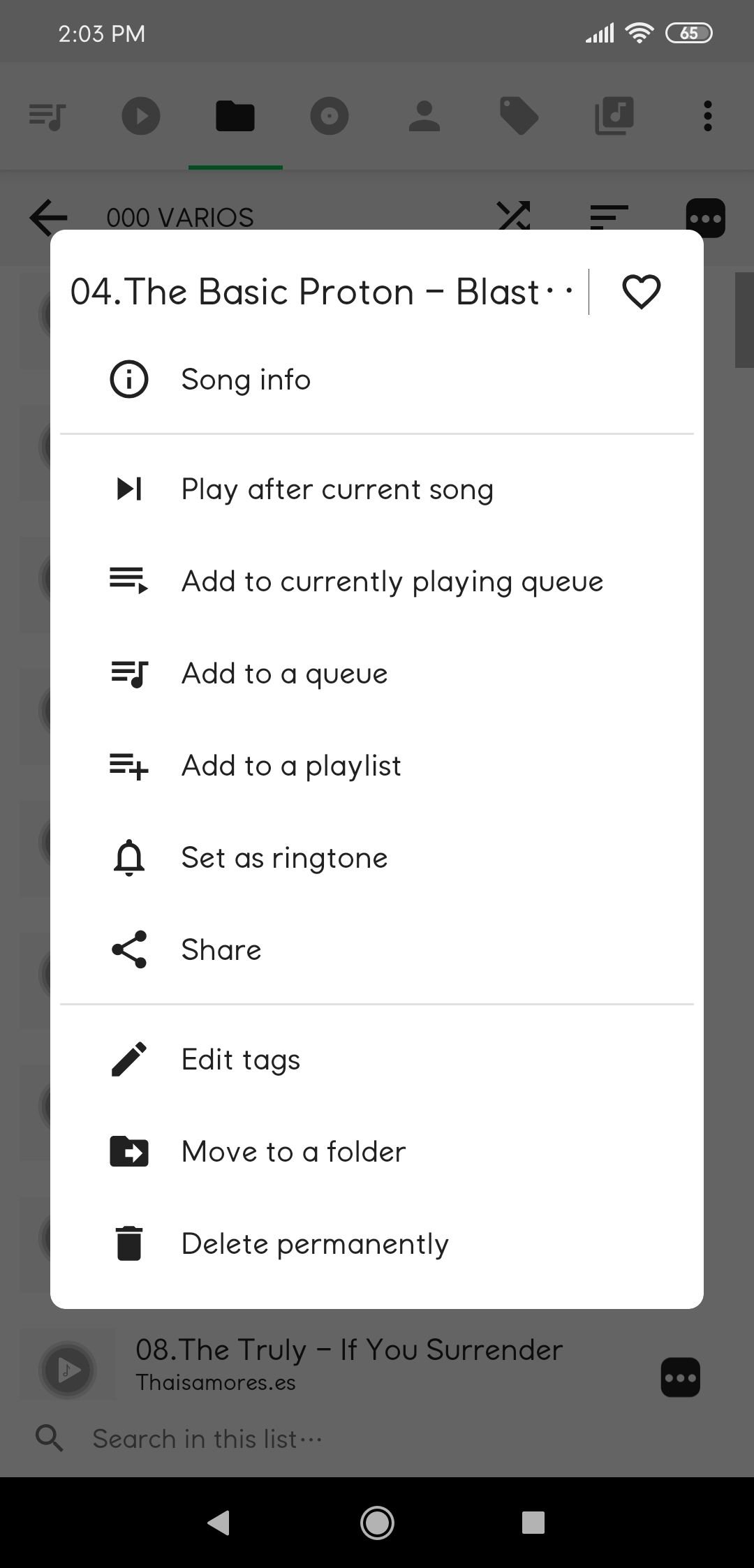The image displays a detailed interface of a music player on a smartphone screen. At the top, a medium gray background header features the time, "2:03 PM" on the left. To the right, full data signal bars and Wi-Fi service are indicated, along with a battery status icon showing "65%" in an oval with a white border.

Beneath this is a white header area containing several icons. On the left, there is a music note icon, followed by a play icon, and a folder icon that is marked as selected with a black color and a green underline. Moving right, there is a thick gray bordered circle, a user icon, a tag icon, another music note icon, and finally, three black dots representing a dropdown menu.

An overlay notification or submenu appears in the top-left corner of the screen. It reads "04. The Basic Proton - Blast" followed by two spaced dots. A faint gray line divider separates this from a heart icon on the right side, which allows the user to like the song. Below the heart icon, there is an eye icon encircled, next to the text "Song Info," followed by another gray line divider.

Multiple actionable options are listed underneath: "Play After Current Song," "Add to Currently Playing Queue," "Add to a Queue," "Add to a Playlist," "Set as Ringtone," and "Share." At the bottom, there's another divider with the last three options: "Edit Tags," "Move to a Folder," and "Delete Permanently."